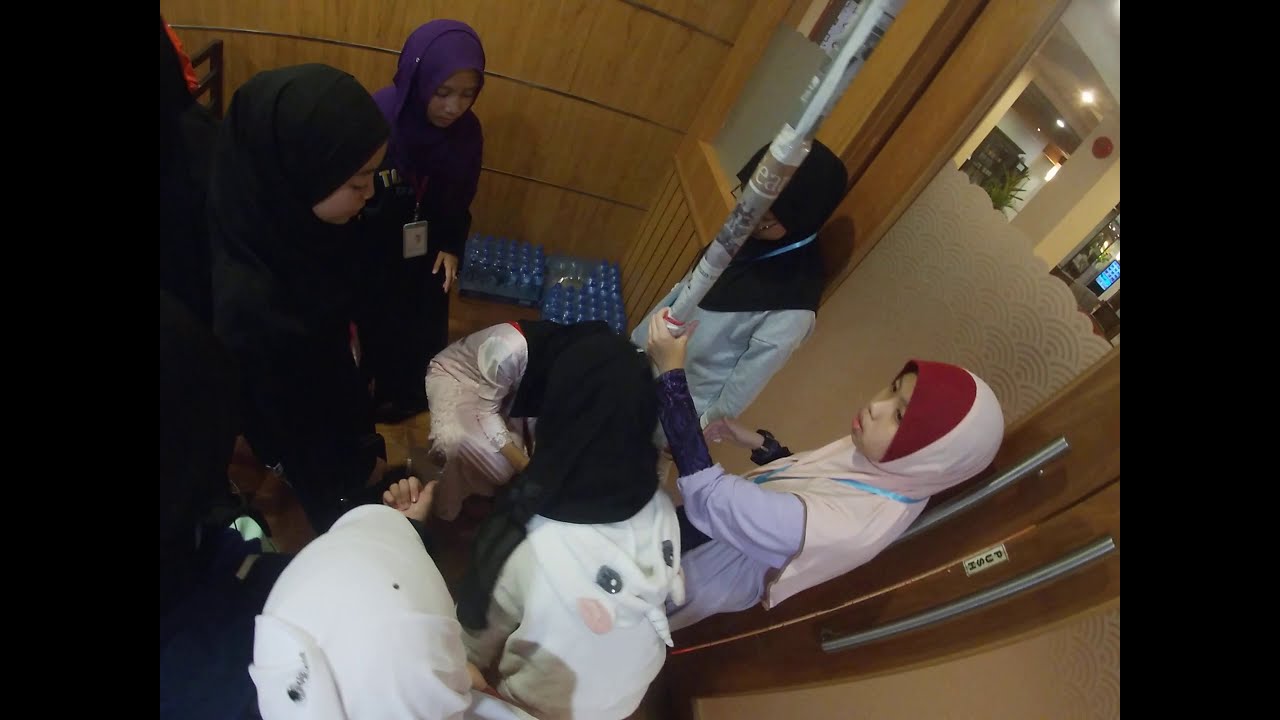This full-color photograph, taken indoors from a slightly elevated angle, captures a small, well-lit, wood-paneled room with black vertical bars framing the left and right of the image. The scene features a group of predominantly young Muslim women and girls wearing hijabs and long outfits, suggesting an Asian descent. They are gathered around one woman kneeling on the floor, with what appears to be a pole wrapped in newspaper in her hands. To the side, cases of bottled water are stacked against a brown-paneled wall, next to a bench where some of the women are seated. A unique detail includes one individual in a hoodie designed with the face and horn of a unicorn. The background reveals a pair of double doors with large metal handles labeled “push,” leading to another well-lit room adorned with plants and a TV or video screen.